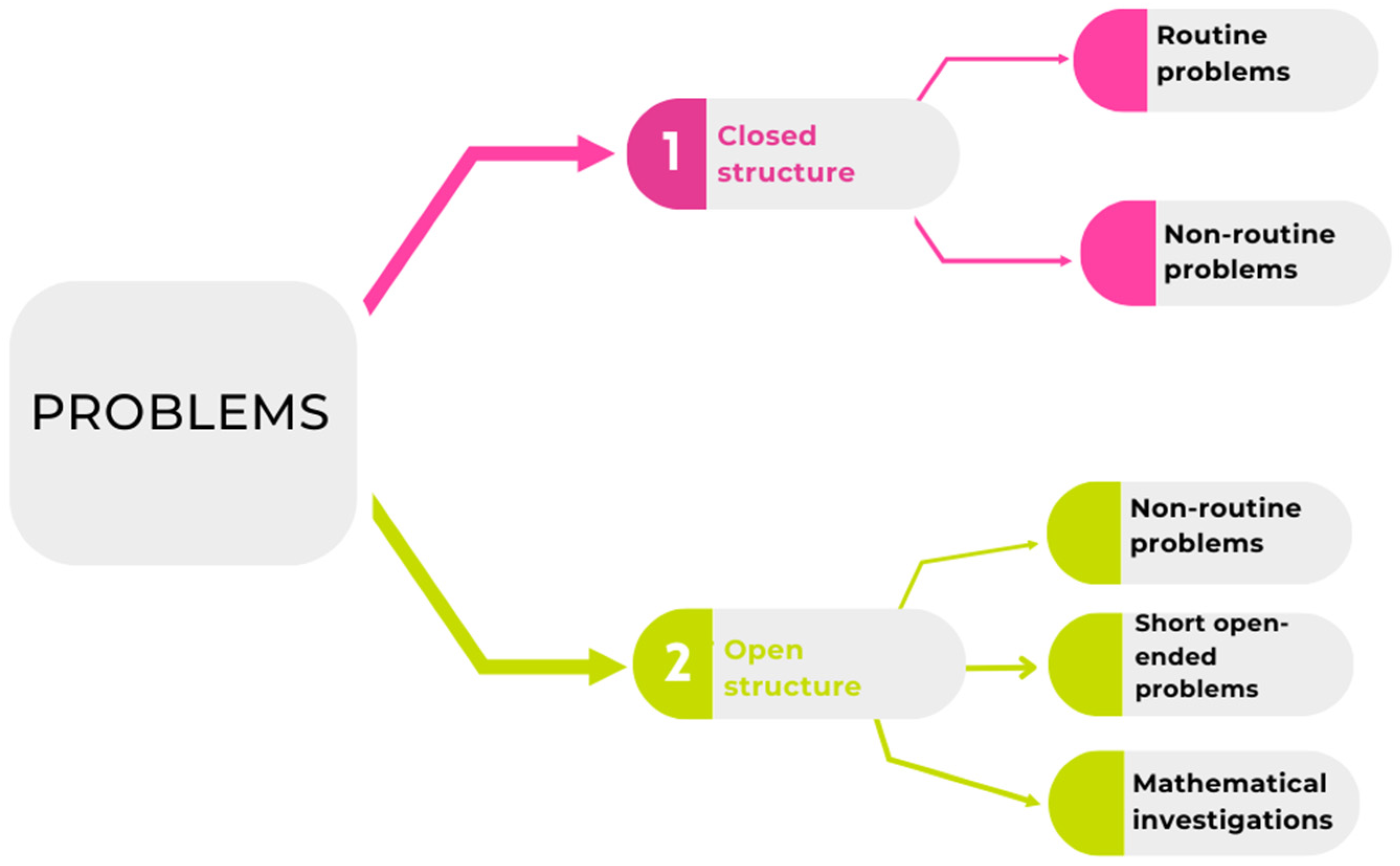The diagram features a structured layout on a white background. On the left side, a light gray square labeled "Problems" in black text serves as the starting point. Two arrows extend from this square to the right: a pink arrow at the top labeled "1. Closed Structure" and a green arrow at the bottom labeled "2. Open Structure."

From the "Closed Structure," pink arrows branch off to two ovals. The top oval is labeled "Routine Problems," and the bottom oval is labeled "Non-Routine Problems," both having a gray background with black text and a pink strip.

From the "Open Structure," green arrows extend to three ovals. The top oval says "Non-Routine Problems," the middle oval says "Short Open-Ended Problems," and the bottom oval says "Mathematical Investigations." These ovals also have a gray background with black text and a green strip. Each element clearly delineates the types of problems and their respective structures, making the relationships and categories easily distinguishable.